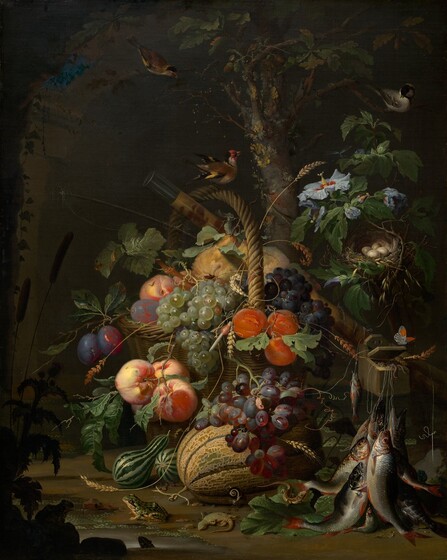In this digital painting, a dark and detailed vignette unfolds, centered around an assortment of food items and wildlife beneath the shadowy canopy of a tree. Nestled against the tree trunk are clusters of fruits, including red and green grapes, plums, nectarines, and peaches, all depicted with rich, saturated hues that stand out against the somber background. A basket to the left brims with more round fruits like plums, subtly hinting at the variegated bounty within. 

Below the vibrant produce, a green-and-gray squash and a couple of gourds peek out, adding texture to the composition. To the right, a hook dangles about five or six fish, meticulously portrayed to emphasize their sleek forms. Near this arrangement, a small nest cradles a few eggs, evoking a moment of delicate stillness in the otherwise abundant scene. 

Adding a touch of liveliness, a frog sits on the forest floor and a chicken balances on a rope near the top of the tree, their presence accompanied by the slight rustle of foliage. Further up in the branches, two birds quietly observe the tableau below. The painting's dark background creates an almost mystical atmosphere, where an archway on the left frames the scene in a subtle hint of another world beyond.